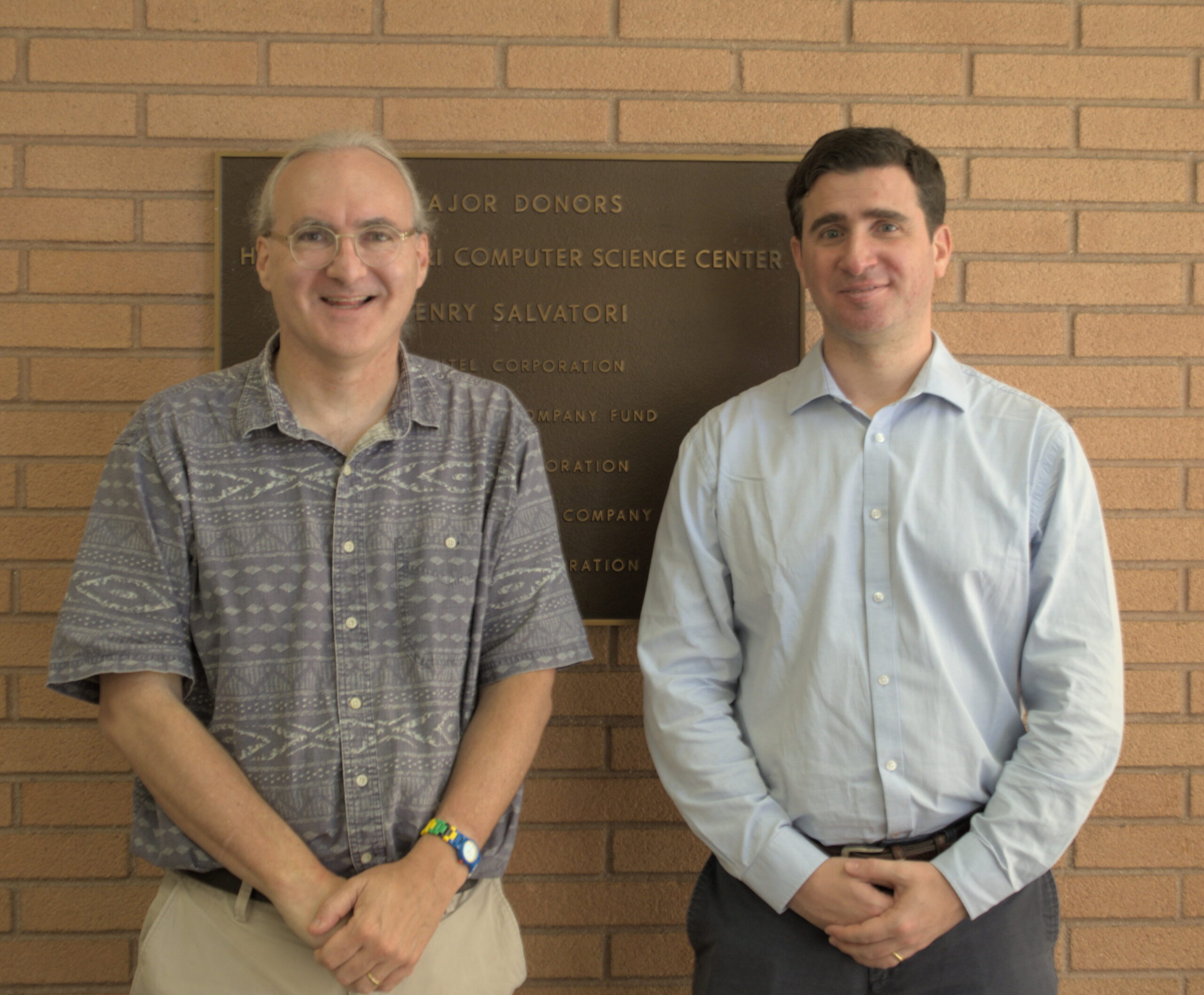This is an image of two men, possibly related due to their similar facial features, standing side by side with their hands folded across their waists. They are positioned in front of an orange-tan brick wall adorned with a brown plaque that partially reads "Computer Science Center," along with the name "Henry Salvatore." The plaque mentions major donors, though some text is obscured.

The man on the left is middle-aged with long hair pulled back, revealing his forehead. He wears clear round glasses and smiles openly, showing his upper teeth. His outfit includes a short-sleeved gray patterned shirt, featuring horizontal stripes and diamond shapes, and gray khaki pants held by a belt. He accessorizes with a beaded watch band in blue, yellow, and green, along with a wedding ring.

The younger man on the right has short brown hair and a faint smile. He is dressed in a light gray button-up shirt with long sleeves and dark gray pants, also secured by a belt. Like the man on the left, he wears a wedding ring. Both men stand calmly in front of the distinguished plaque, hinting at a connection to the Computer Science Center.